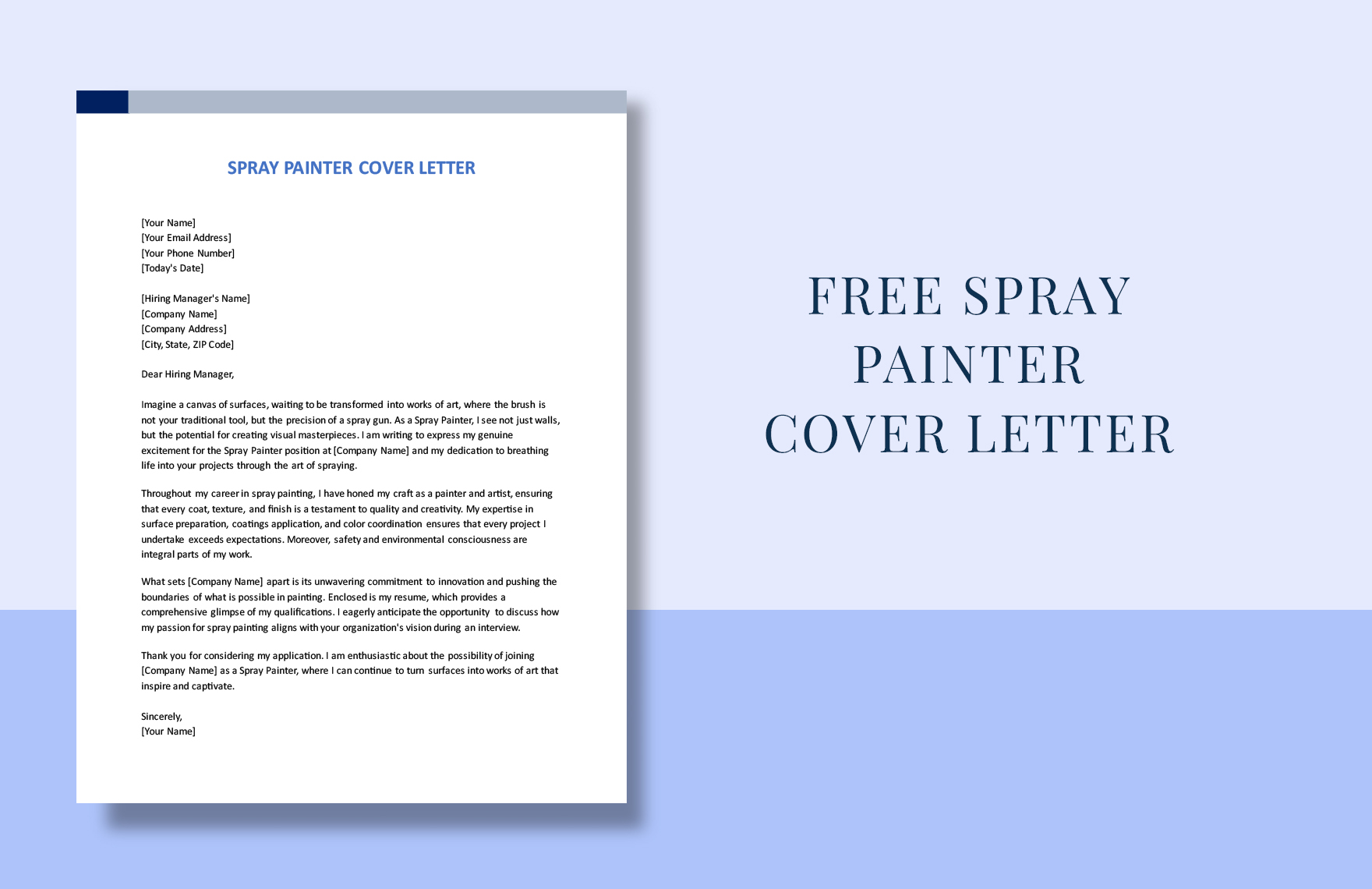This image is a digital mock-up designed to present a free spray painter cover letter template, featuring detailed design elements and examples of placeholder text for customization. The background is composed of two blue rectangles: the top three-fourths of the image is a light blue, while the bottom one-fourth is a darker blue. On the left side of the image, there's an overlaid cover letter template which is displayed on a white sheet of paper. At the very top of this sheet, there's a short blue rectangle in the upper left corner and a long gray rectangle extending across the remainder of the top section. The heading on the paper reads "Spray Painter Cover Letter" in blue, capitalized text, and below it, there's placeholder text in very small black font that is too minute to read fluently.

This cover letter template includes brackets for entering your own personal information such as your name, email address, phone number, today's date, hiring manager's name, company name, company address, city, state, and zip code. The body of the letter begins with, "Dear Hiring Manager," and an example introductory phrase that reads, "Imagine a canvas of surfaces waiting to be transformed into works of art, where the brush is not your traditional tool but the precision of a spray gun. As a spray painter, I see not just walls but the potential for creating visual masterpieces. I'm writing to express my genuine excitement for the spray painter position at [Company Name] and my dedication to breathing life into your projects through the art of spraying."

On the right side of the image, in darker text, it prominently states "Free Spray Painter Cover Letter," reinforcing that this is a sample template available for use. The overall presentation looks similar to a slide for a presentation or an advertisement for the cover letter template, aimed at guiding users to create professional and personalized cover letters for spray painter job applications.